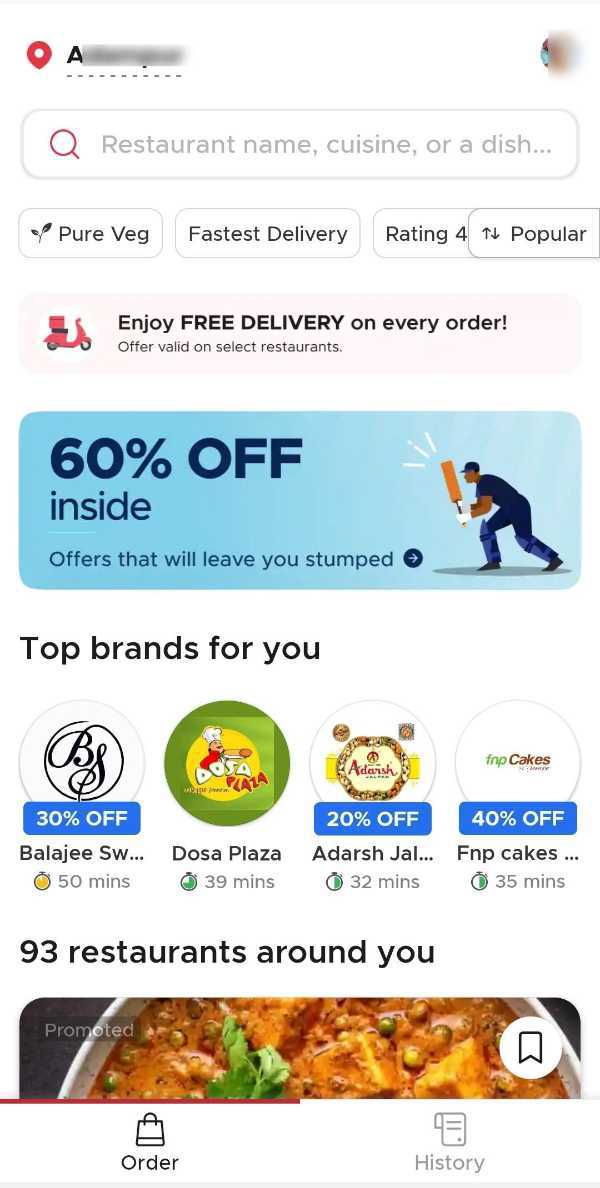Screenshot of a restaurant search feature on a smartphone:

The image captures a smartphone screen displaying an app interface for searching restaurants. At the top, the user’s profile photo is visible next to the app name, which is highlighted. Below this, an icon indicating the user's location is present, followed by a prominent search bar reading "Restaurant name, cuisine, or a dish."

Just beneath the search bar, there are several filter tabs: "Pure Veg," "Fastest Delivery," "Rating 4+", and "Popular," indicated by up and down arrows. 

The interface features a banner with an image of a scooter, advertising "Enjoy Free Delivery on Every Order!" marked with an exclamation point, and specifying that the offer is valid on select restaurants.

Following this is another promotional banner offering “60% Off!” accompanied by the slogan "Offers That Will Leave You Stumped," illustrated with an image of a cricket player in full gear holding a bat.

Further down, the section titled "Top Brands for You" showcases various restaurants and their respective offers and estimated delivery times: 
- "Belaji" with 30% off and a 50-minute delivery time,
- "Dosa Plaza" offering 20% off with a 39-minute delivery time,
- "Adarsh" providing 20% off and a 32-minute delivery time,
- "FNP Cakes" offering 40% off with a 35-minute delivery time.

The app indicates there are "93 Restaurants Around You." Below this, there is an image of a promoted meal or restaurant, partially cut off, featuring a circular bookmark icon.

At the bottom of the screen, two tabs are available: one for "Order" and another for "History."